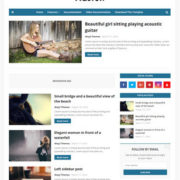The image in question is a blurry screenshot, appearing to be from a web page that does not conform to standard widescreen dimensions; it is slightly taller than it is wide. The dominant color scheme is a white background. Along the left side of the webpage, there are several images with bold black text adjacent to them, presumably describing either the images themselves or the stories associated with them. Beneath this bold text, there are smaller text blocks that are illegible. A large blue rectangular button, likely a "Read More" call-to-action, is also present but its text is indiscernible.

The most prominent image features a young blonde woman seated outdoors against what appears to be a wooden barn. She is positioned on the grass next to a large pile of wood. She has an acoustic guitar in her lap, balanced on her right thigh, with her right hand strumming and her left hand forming a chord. This specific image is accompanied by the caption, "Beautiful girl sitting playing acoustic guitar," suggesting that it is more focused on the image rather than an accompanying story. The remaining images are smaller and less discernible, with their details obscured in the blur.